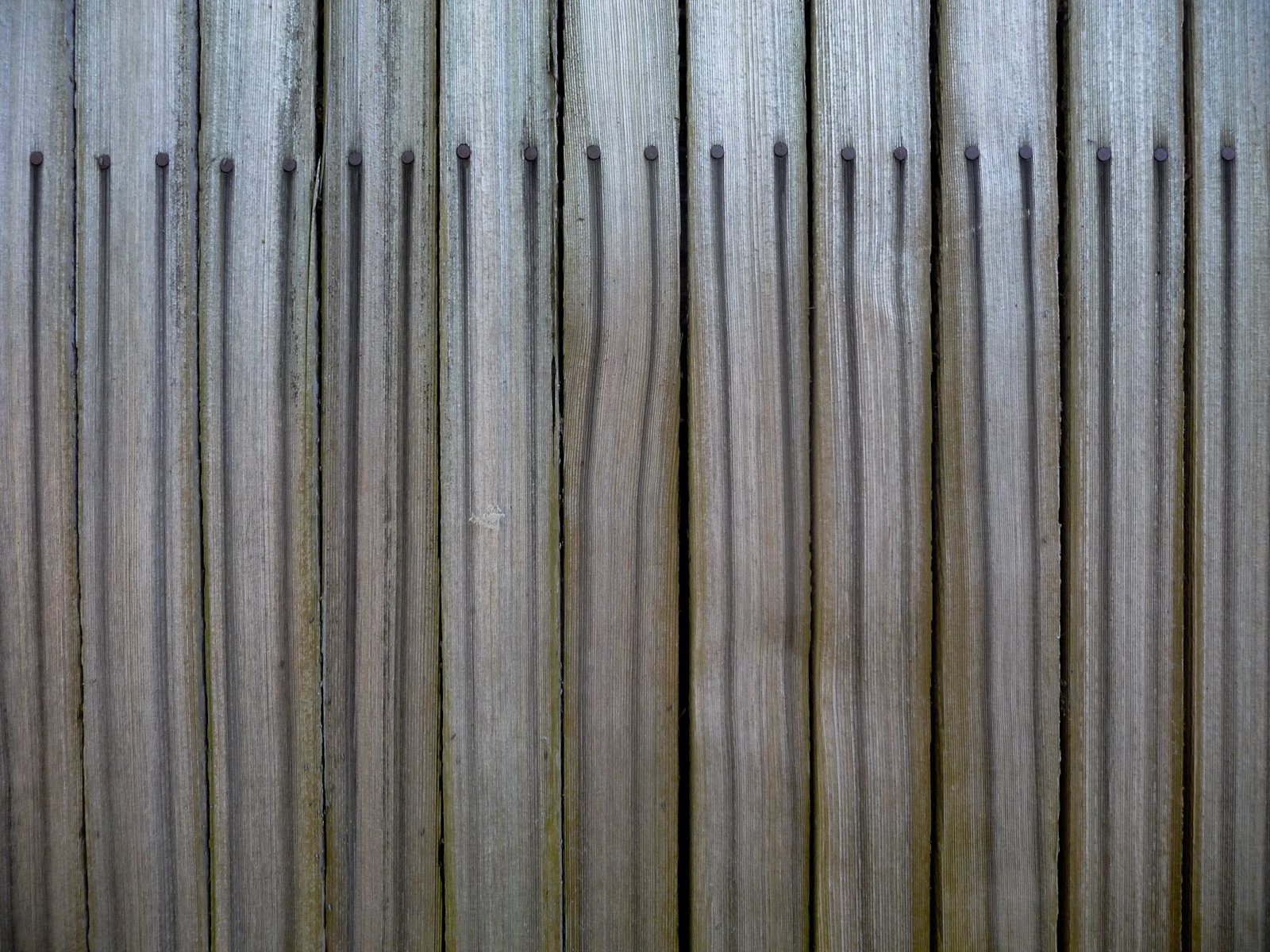This image showcases an aged wooden fence comprised of 11 vertical slats. Each of these skinny, grayish wooden posts exhibits noticeable signs of wear and weathering, with black streaks running from top to bottom. The grain of the wood is vividly visible, adding to its rustic appeal. The spacing between the slats varies slightly, with roughly a quarter-inch gap that is particularly noticeable in the middle of the image. Each slat features two black, wavy lines emanating from nails located near the top, tapering off towards the bottom. It's as if rainwater has caused these black lines to streak and fade progressively down the posts, adding to the weathered, antique look of the fence.